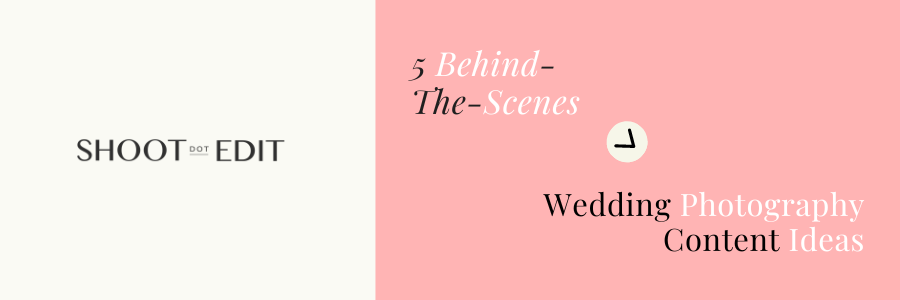The image is divided into two sections, side-by-side. On the left, the background is white with black, uppercase text that says "SHOOT" and "EDIT," with a smaller, gray dot in between the words that has an underline. The right section features a pink background with mixed font text. It reads "5 Behind the Scenes" in italicized, white letters, and has a downward-pointing arrow inside a white circle. Below the circle, in black and white text, it says "Wedding Photography Content Ideas." This visually cohesive image serves as a guide to generating content ideas for wedding photography, emphasizing behind-the-scenes insights.